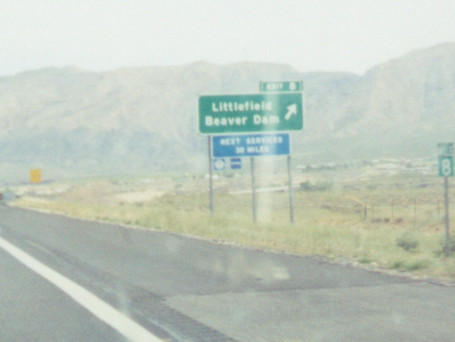The photograph, taken during the daytime from inside a car, captures a view of a highway through the windshield. In the bottom left corner, the gray surface of the highway is bordered by a white line marking the lane's edge. To the right of the highway, there is a light green grassy area. Prominently featured on the right side of the image is a series of three vertical gray posts holding three signs. The top sign is a small green rectangle indicating "Exit 8." Below it, a larger green sign reads "Littlefield Beaver Dam" with an arrow pointing up and to the right. The bottom sign, a blue rectangle, partially visible and slightly blurred, likely mentions rest services available in 30 miles. In the background, a range of flatter hilltops or mountains lies under a light blue sky, adding a scenic backdrop to the image. The overall lighting is somewhat washed out, giving a slightly muted appearance to the photograph.